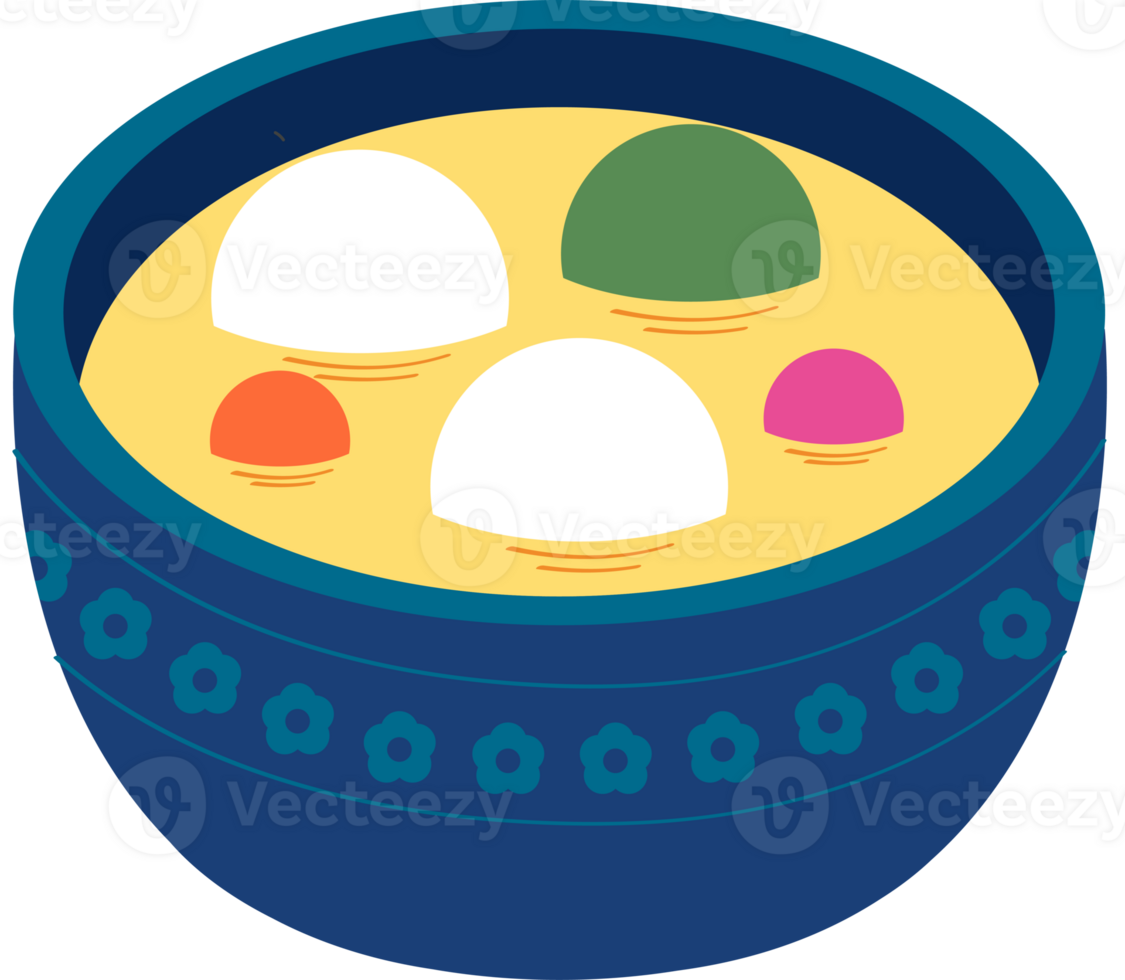This detailed cartoon image depicts a navy blue bowl adorned with a pattern of frosted, hollow-centered flowers encircling the rim. Inside the bowl, a vibrant yellow broth fills the space, contrasting with the blue exterior. Floating on the surface are five dome-shaped objects, partially submerged. Three of these are large, with two being white and one a forest green. Additionally, there are two smaller domes, one orange and one purple, adding a splash of color to the scene. The entire image is set against a plain white background and repeatedly features the watermark "Vecteezy" across its surface.